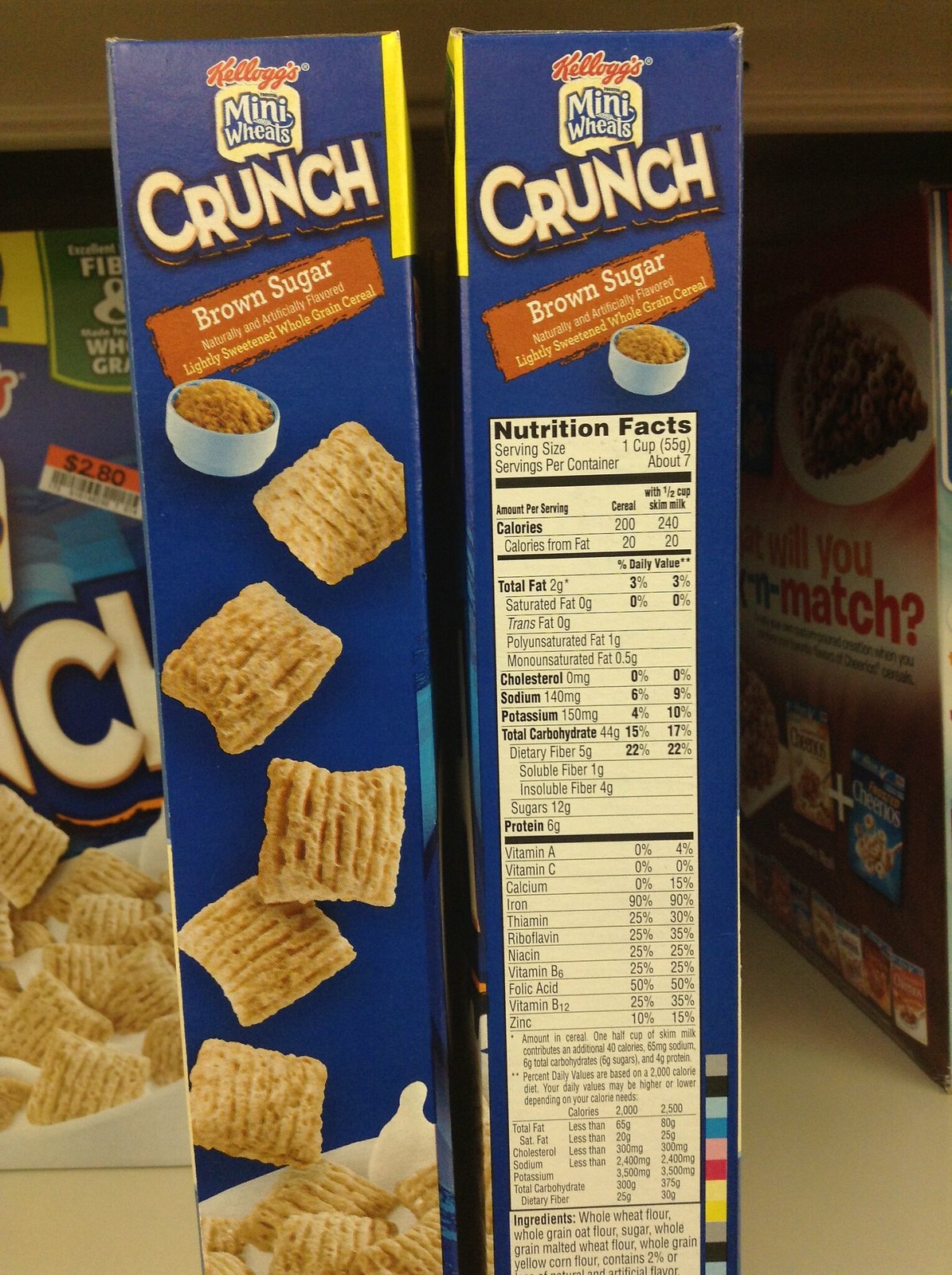The photograph captures two Kellogg's Mini Wheats Crunch cereal boxes positioned side by side, showing primarily their side views against a blue background with white writing. At the top of both boxes, the red Kellogg's logo is clearly visible. Below it, an image resembling a piece of toast has the word "Mini Wheats" on it, and beneath that, in large white letters, is the word "Crunch." There is an orange banner near the bottom stating "Brown Sugar" in white letters.

On the left box, there are visual examples of the cereal — small, square-shaped pieces resembling Chex, which appear to be floating into a bowl of milk, suggesting their crunchy texture and flavor. A separate close-up image on the box shows a white bowl filled with what looks like brown sugar. 

The right box prominently features a white rectangular panel that contains the nutrition facts, listing vital information such as fat, cholesterol, salt, and total carbohydrate content, along with serving suggestions and recommended daily allowances. This panel also highlights the healthy ingredients within the cereal. Below the nutrition panel, additional items are depicted, though their specifics are not clear.